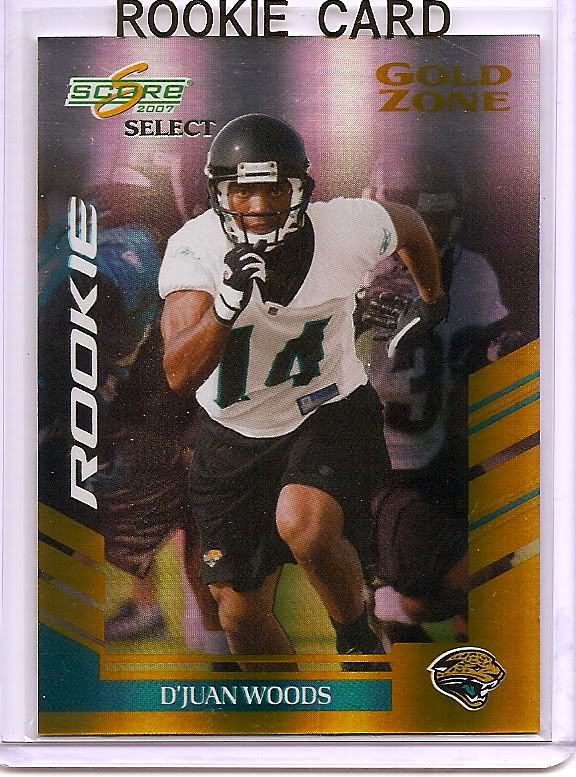This image features a rectangular, white-bordered card prominently displaying a mid-action photograph of an American football player. The player, identified as Dijon Woods, is captured running towards the front of the image. He is dressed in a football uniform, which includes a black helmet, black and white gloves, a white jersey with the number 14 on the chest, and short black pants. In the background, other football players can be seen, although they are slightly blurred to emphasize the main subject. 

Text details are strategically placed around the card: at the top left corner, "Score 2007 Select" is printed, while the top right corner reads "Gold Zone Kaohsiung." Along the left side, the word "Rookie" is displayed, and at the bottom, "Dijon Woods." The bottom right features a detailed drawing of a tiger's face. Additionally, the top edge of the card includes the label "Rookie Card."